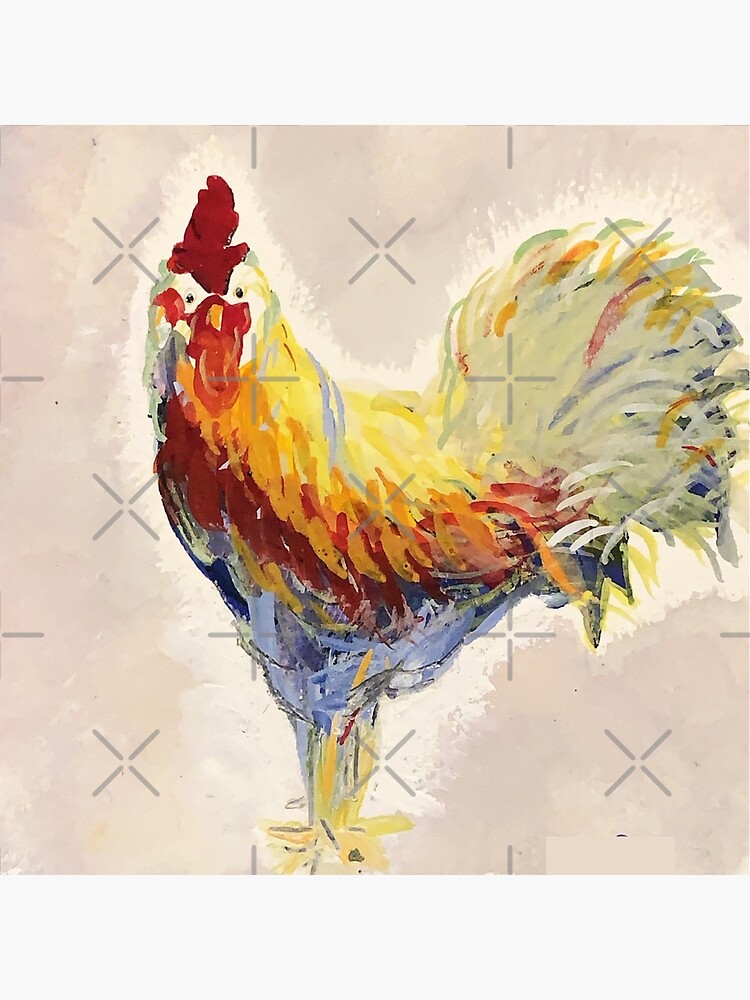This detailed impressionistic painting depicts a vibrant rooster set against a light grey background, with the focal image framed within a square. The main backdrop of the painting consists of a blend of light brown and beige splotches, overlaid with interspersed grey lines forming X and plus sign patterns. These patterns are systematically arranged across the image.

The rooster itself is painted with meticulous attention to color and detail. It stands with its body oriented to the left while the head is turned to face forward, engaging directly with the viewer. Bold colors define its form: its feet are a striking yellow, transitioning upward to a blue underbelly marked by light and dark blue tones. The chest showcases a deep red hue, progressing to an orange stripe, then a yellow stripe, creating a layered, rainbow-like effect on its torso. The head is outlined in sand green with a white face adorned by a dark red comb, dark yellow to orange beak, and small black eyes.

The rooster's tail feathers display a rich mix of sand and olive green, accented with a slightly yellow outline on top and a blue outline at the back. Surrounding the rooster is a subtle white halo that blends seamlessly into the background splotches, enhancing the figure's prominence in the composition. The artwork's folk art style is evident through its use of simple, yet vivid color schemes and the stylized representation of the rooster. This image also contains a watermark, suggesting it might be a reproduction or digitally protected piece.